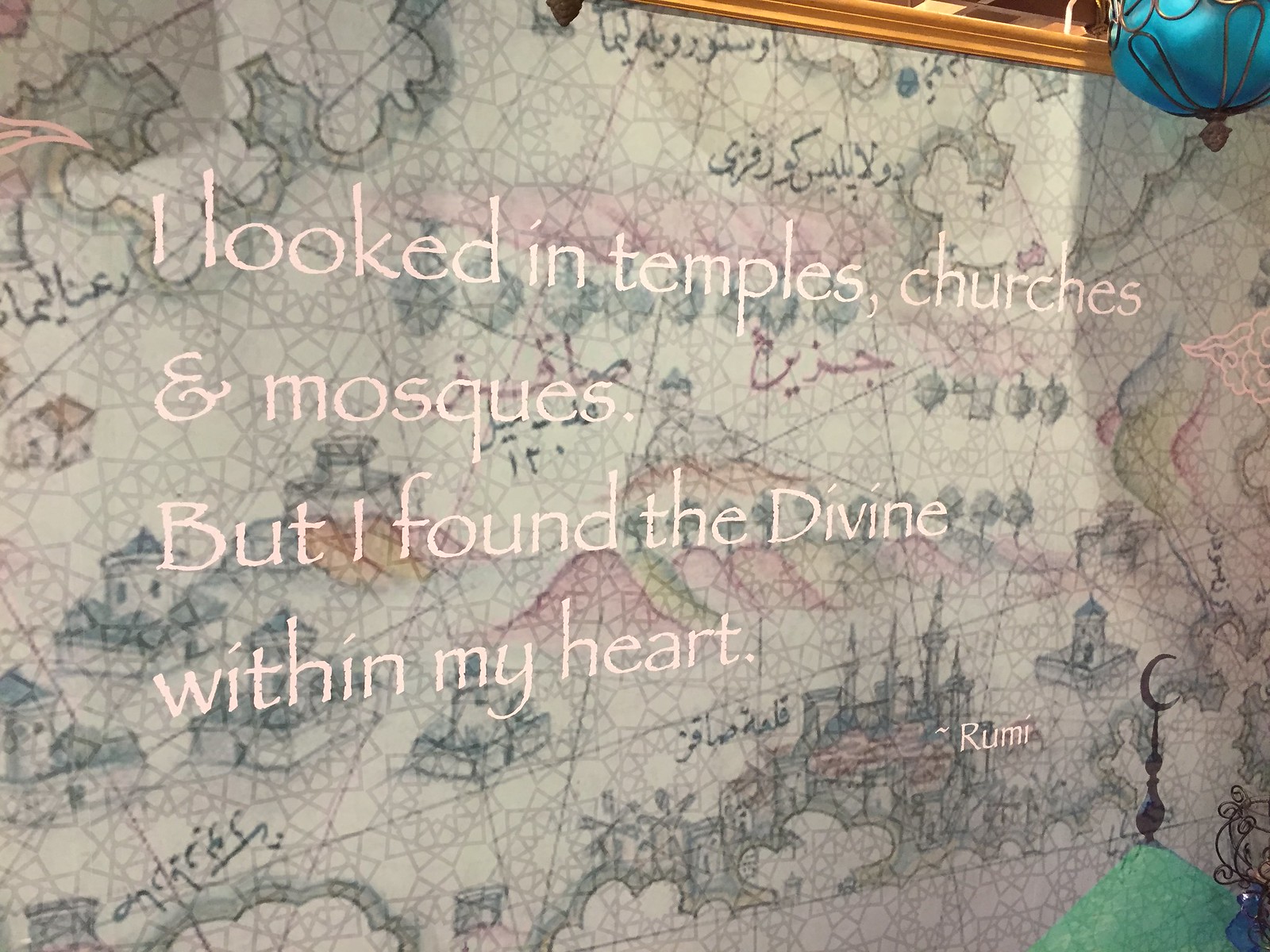The image showcases a white background adorned with a variety of geometric shapes, such as triangles and rectangles, in grayscale hues. Over these shapes, there are detailed illustrations of small huts, castles, rolling hills, and clouds. Integrated within the artwork are snippets of text that appear to be in Arabic script, adding an extra layer of complexity and cultural context.

At the top of the image, in digitally added white text, is a poignant quote by the poet Rumi: "I looked in temples, churches and mosques, but I found the divine within my heart." This quote overlays the artistic elements, serving as a focal point. To the top right of the image, there is a peculiar blue, bulbous object that resembles a lantern or an ornate decoration, adding a touch of mystery to the overall composition.